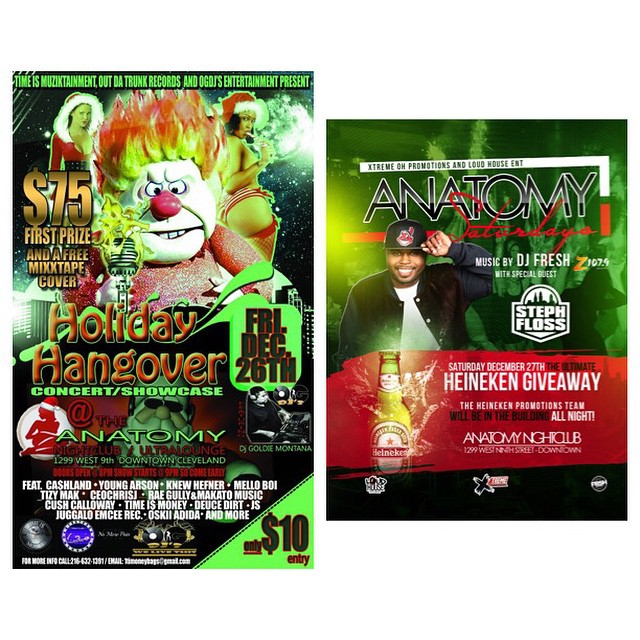The image features two detailed flyers for Anatomy Nightclub side-by-side, both promoting different events. The flyer on the left, which is longer and thinner, showcases the "Holiday Hangover Concert & Showcase" event scheduled for Friday, December 26th. Dominating the top section is a cartoonish, evil clown face with flaming green hair, green writing, and a menacing grin. Flanking the clown are two Santa-clad women—one in a full Santa outfit on the left and one scantily dressed with a Santa hat and red fishnet stockings on the right. The clown's body is emblazoned with the event name, "Holiday Hangover," in bold red font, with "Friday, December 26th" and performer credits beneath it. The bottom right corner highlights a $10 entry fee and mentions a $75 first prize coupled with a free mixtape cover.

The flyer on the right has a green background transitioning to black towards the bottom. It prominently displays the Anatomy Nightclub's name at the top. To the left is an image of a young African American man wearing a Cleveland Indians hat and a white t-shirt under a black long-sleeve jacket, raising his left hand to the brim of his hat. Further down, a red splotch announces a Heineken giveaway featuring a picture of a Heineken bottle, emphasized with white text. The flyer also states music will be by DJ Fresh with a special guest appearance by Steph Floss, indicating another event taking place on Saturday, December 27th.